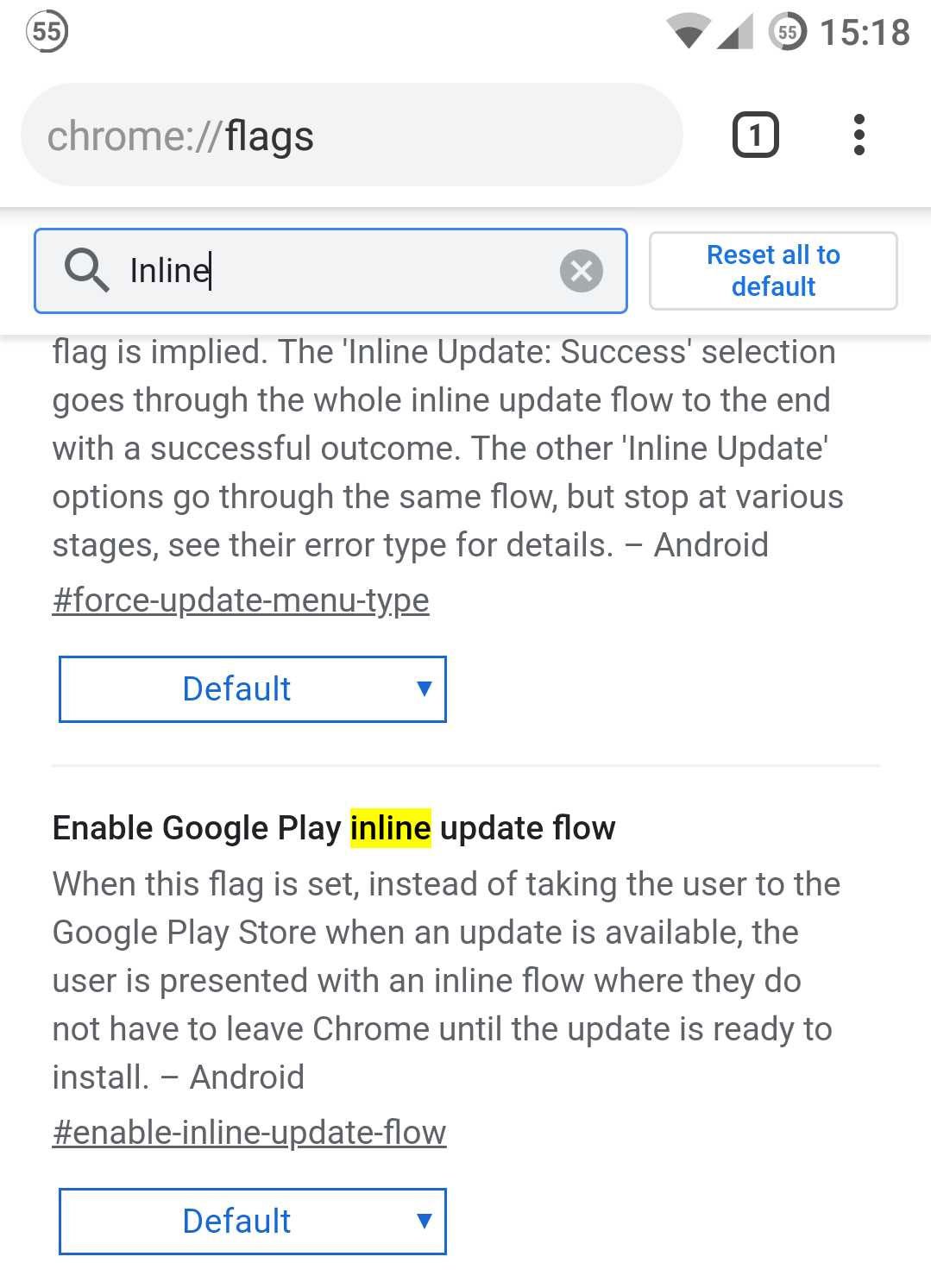The image features a white background with the following details:
- At the top, there is a circle with "55" inside, accompanied by the notation "1518".
- Below that, a blue box contains the word "Chrome", followed by two dashes (--), and flag icons. 
- There's also a number "1" next to a small black square, and a cluster of three black dots.
- A line separates this from another blue box that states "Inline", with a small "X" at the back.
- A button labeled "Reset All to Default" is present.
- Text in the image explains that setting the "Flag is implied" option will ensure the "Inline update success selection" goes through the full inline update process to completion. Other inline update options follow a similar flow but stop at various stages, with error types described in detail for Android.
- The text also mentions "hashtag force update menu type" which is underlined.
- Another blue box, white on the inside, displays the word "Default" in blue, accompanied by a down arrow.
- The phrase "enable Google Play inline update flow" is highlighted with a yellow square around "inline".
- Further text explains that when this flag is set, instead of directing the user to the Google Play Store for available updates, the user experiences an inline flow, staying within Chrome until the update is ready for installation. This information applies to Android.
- A hashtag "enable inline update flow" is underlined.
- Finally, a "Default" button is shown, with the text "Default" in blue on a white button outlined in blue, with a blue down arrow.